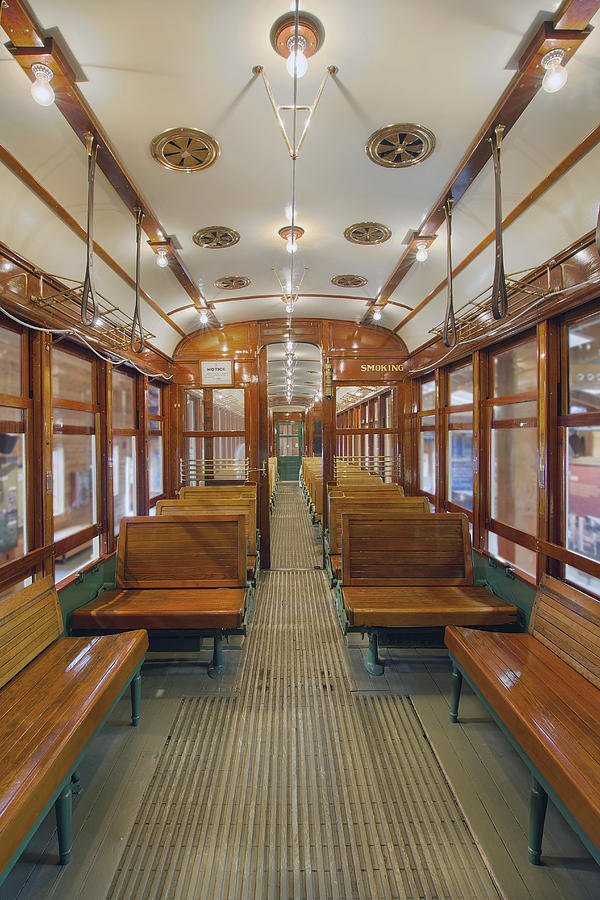This photograph showcases the interior of an old, possibly museum-displayed train car, bathed in the rich tones of polished dark and light brown wood. The train car is entirely empty, allowing a clear view down the center aisle to the back of the car. Rows of wooden benches, featuring green legs, line either side of the aisle, with both seating and backrests crafted from wooden boards. The floor sports a gray, grated look, enhancing the rustic charm. Golden vent covers run along the ceiling's center, with old-fashioned light bulbs providing illumination. The ceiling itself is primarily white, intersected by multiple wooden bars forming a rectangular pattern. Brass luggage racks hover above the seats and small loops hang from the ceiling, offering stability for standing passengers. Large windows encircle the car, revealing indistinct views outside, grounding the scene in a sepia-toned nostalgia.